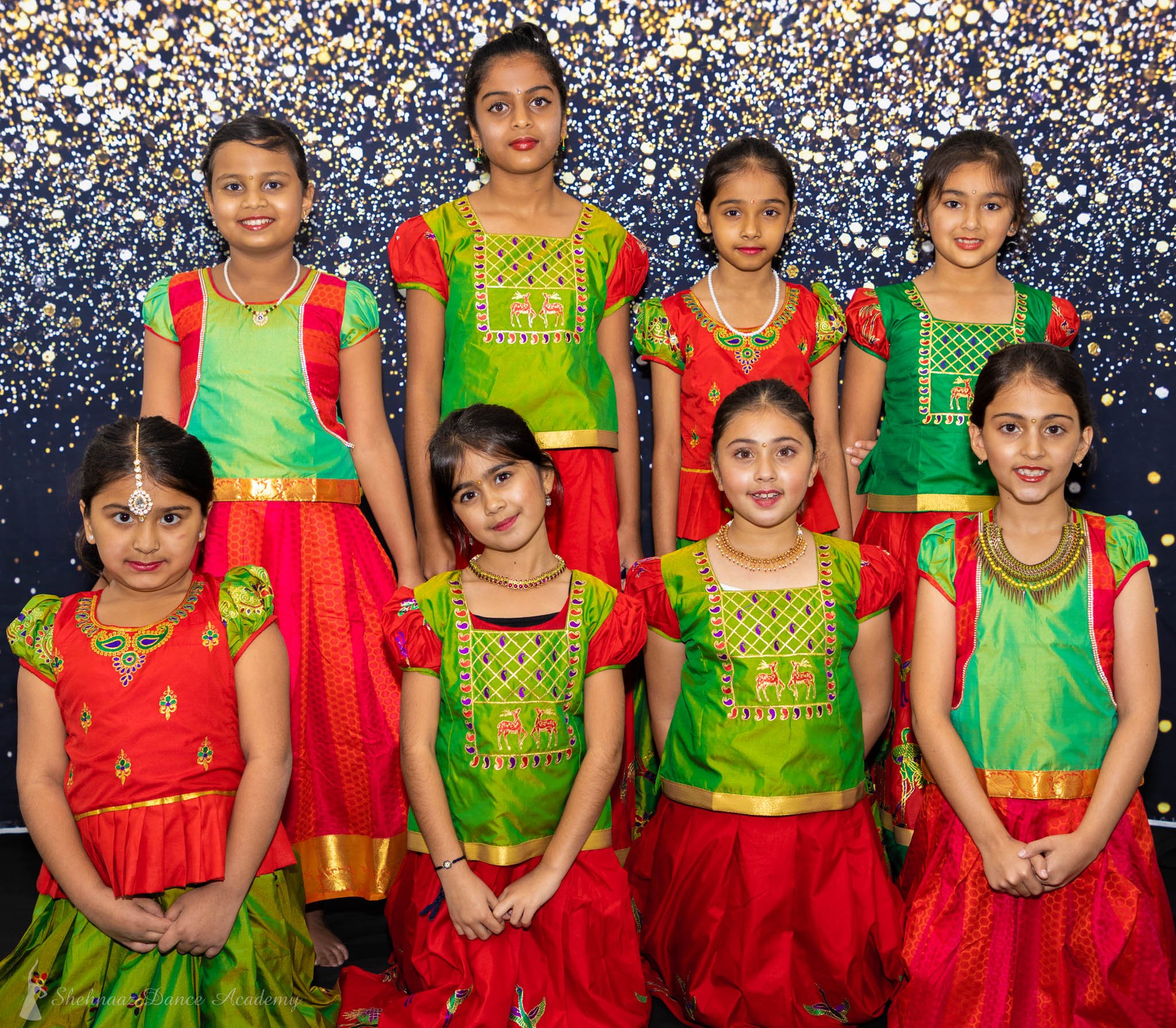This is a photograph of eight young girls, likely of Indian or Southeast Asian descent, dressed in vibrant red and green costumes. Some of the girls wear green tops paired with red bottoms, while others wear red tops with green bottoms. They are arranged in two rows with four girls standing in the back and four kneeling in the front. Their dark hair and happy smiles are striking, with most girls looking directly at the camera, exuding joy. Notably, the girl on the bottom left sports a traditional forehead jewelry accessory. The background features a dark blue backdrop adorned with golden and silver glittery bubbles, giving a festive and formal feel to the image. This carefully posed photograph suggests they are part of a performing group, possibly dancers, and captures the essence of their cultural attire and cheerful camaraderie.